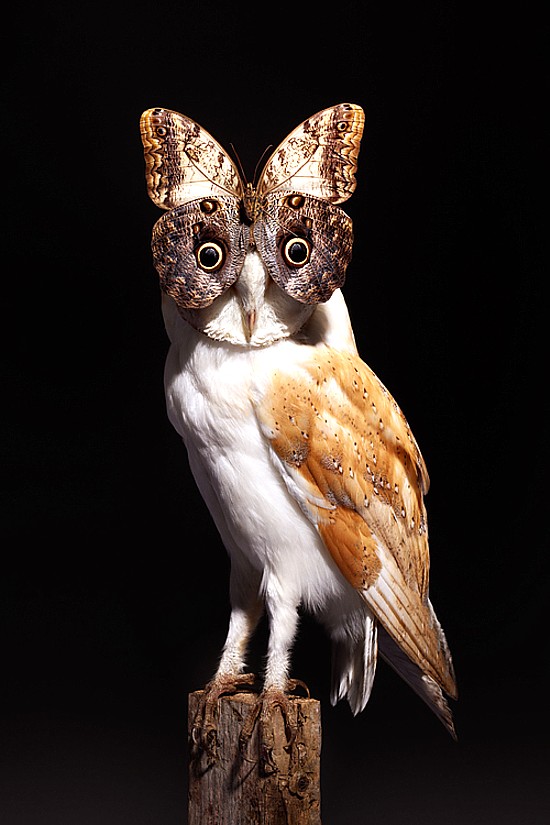This creative digital photograph features an intricately designed owl perched on a tree stump, its talons gripping firmly. The owl, primarily white with touches of tan feathering and brown-tipped wings, presents an unusual and captivating visage. Instead of a typical owl’s face, it showcases an elaborate optical illusion where its eyes and facial features are seamlessly integrated with the wings of a butterfly. The butterfly, with its delicate brown and white patterned wings, covers the owl's face such that the owl's penetrating eyes peer through the butterfly's upper wings. The image is set against a stark black background, which not only enhances the intricate details and contrast of the owl-butterfly hybrid but also draws immediate focus to this surreal and imaginative creature. The overall composition suggests deliberate artistry, most likely falling under the realm of digital creations or photo illustrations, meant to intrigue and mesmerize the viewer.